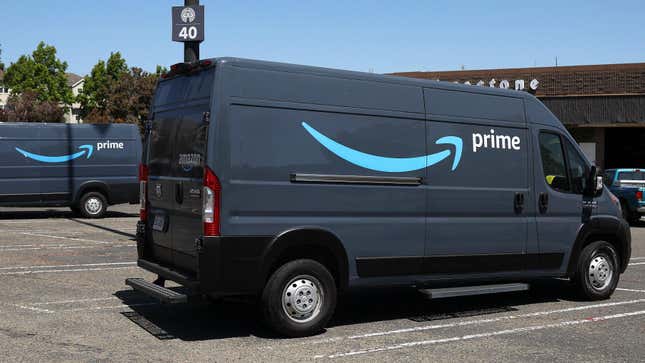The photograph captures a scene in a parking lot in broad daylight, with a clear blue sky overhead. Dominating the foreground is a blue Amazon Prime delivery van, parked facing away from the camera such that the viewer sees the right-hand side of the vehicle. The characteristic Amazon Prime logo, with its blue swooping arrow and “Prime” text, is prominently displayed on the van's side.

In the background to the right, part of a Firestone service center is visible, with the letters "S-T-O-N-E" discernible on its sign, though the full name is obscured by the van. Another Amazon Prime van is situated in the background on the left side of the image, seemingly positioned in the opposite direction with the rear of the truck to the right. However, its logo also faces the same direction as the van in the foreground.

A parking pole marked with the number 40 stands nearby, probably indicating a designated parking spot. The scene epitomizes the ubiquity of Amazon Prime delivery vehicles, underscoring how commonplace such vans have become in shopping center parking lots compared to traditional Postal Service vehicles.